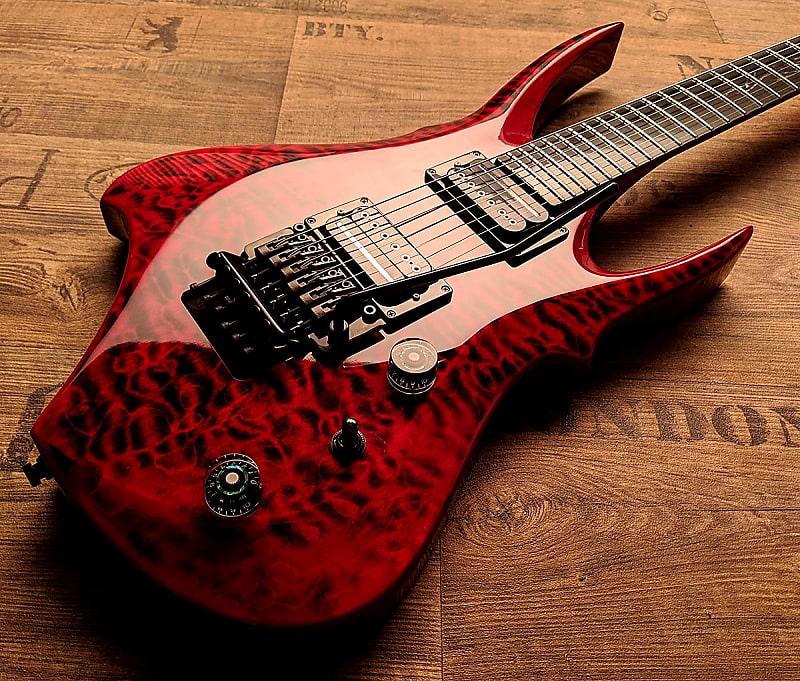The photograph showcases a stylish and premium electric guitar placed on a unique wooden surface. The guitar features a highly polished red body with black wave-like patterns and a light pink center. It is equipped with at least two large black knobs and a small toggle switch situated to the right of the guitar strings. The wooden surface beneath the guitar appears to be made from wooden planks, possibly from transport crates, and is adorned with various burned-in insignias, including a crest with a lion or bear, along with the letters "BTY" and the word "London." The guitar's shadow is cast directly downward, indicating the light source is coming from behind the guitar.